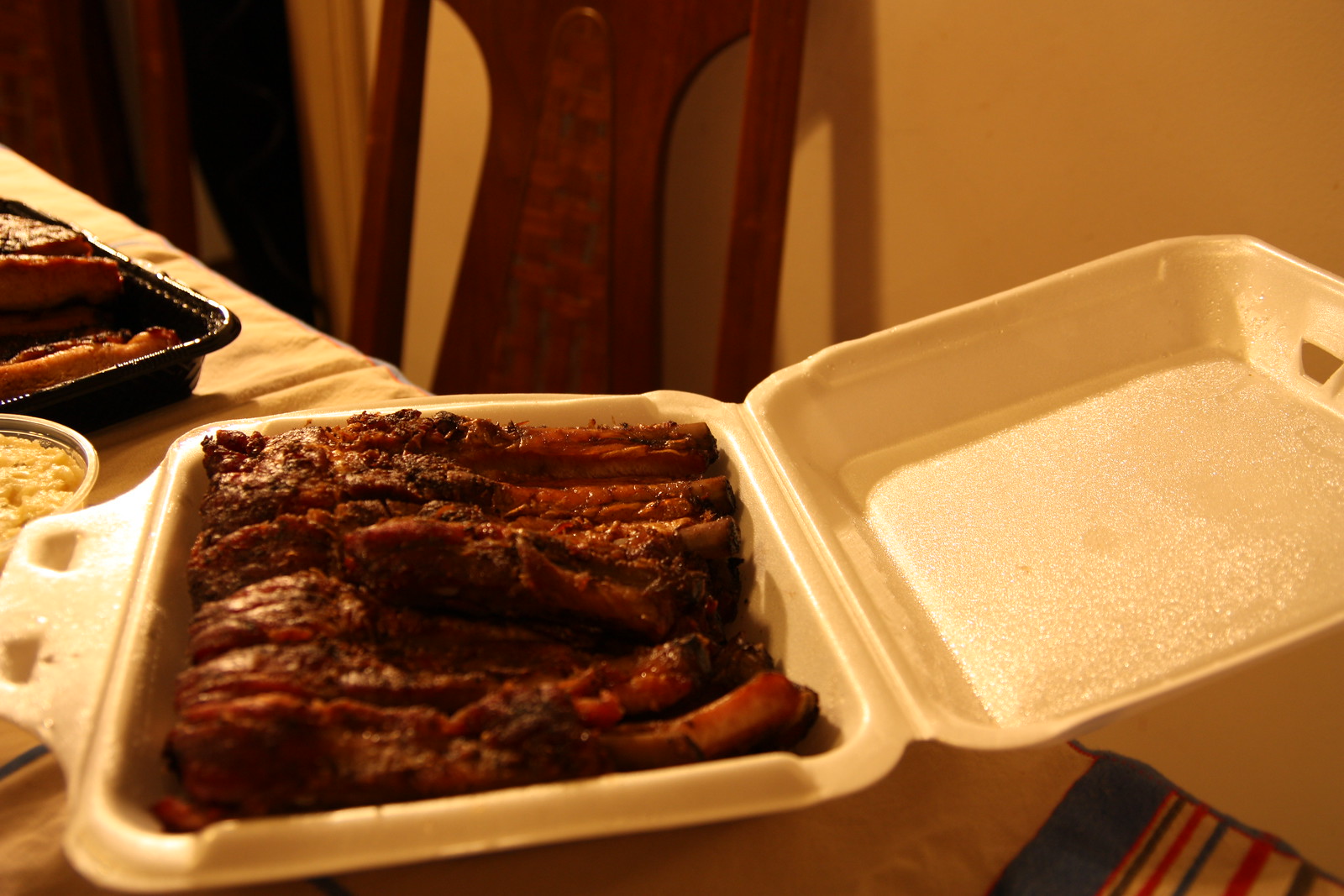In the image, we see a dining setup with a light beige wall in the background, complemented by dark brown wooden chairs framed prominently. The foreground is dominated by a table draped with a yellow cloth, which features intricate patterns with green, black, and red stripes. Diagonally positioned from the upper left to the bottom right, the table also reveals a corner where cloth ends, displaying a small figure with a brown outline.

At the center of this setting lies an open white Styrofoam container filled to the brim with barbecued ribs, likely pork or beef, meticulously arranged in two layers. To the left, another take-out container with a black corner is visible, containing a piece of bread. Adjacent to these containers is a bowl, possibly holding some yellow-hued potato salad, adding more variety to the meal's presentation. This composition highlights the casual, yet hearty, ambiance of a take-out feast enjoyed in a cozy dining area.